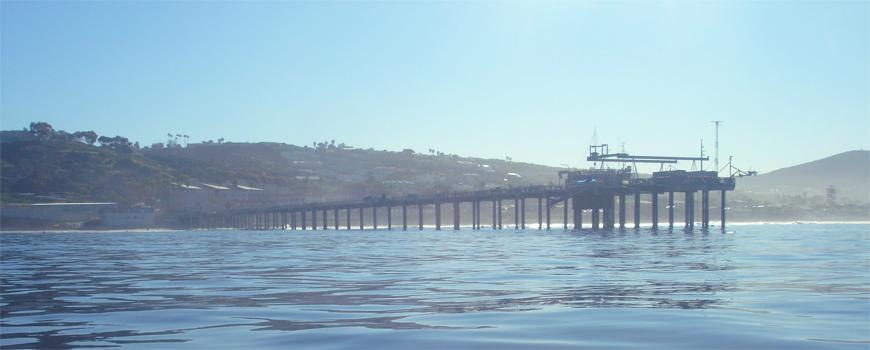The image depicts a serene outdoor scene featuring a vast, slightly wavy ocean occupying the lower half, its deep blue hues interspersed with darker patches. Stretching from the center right and extending leftward over the water, a long pier culminates in a robust metal structure, possibly an oil rig or similar platform, resting on sturdy towers or poles. This elongated deck-like walkway, constructed of wooden planks, leads toward the distant coastline where faint, likely white buildings—potentially hotels, housing, or factories—line the shore. Beyond these structures, the landscape transitions into a lush, green hilly terrain, dotted with trees. To the right side of the image, a prominent green hill rises against the horizon. The entire scene is bathed in sunlight under a clear, azure sky, creating a tranquil and picturesque view.